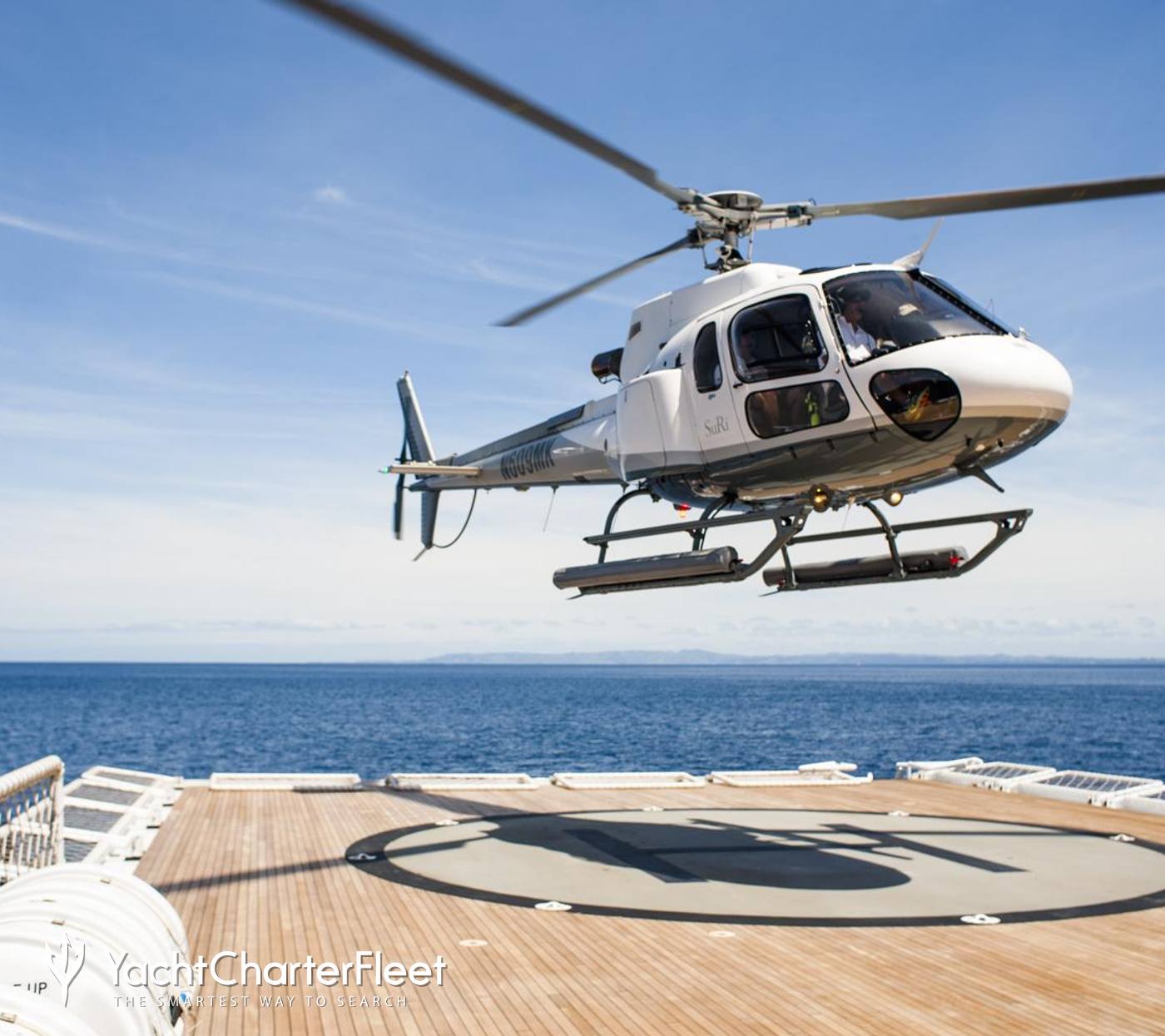In this image, a white helicopter with black spinning blades hovers approximately 10 to 15 feet above a helipad, which is situated on the deck of a large yacht or boat. The helipad features a beige center with a prominent black H enclosed by a black ring. The helicopter, which has a gray stripe wrapping around its front and a dark-colored bottom, appears to be either landing or taking off. The setting is serene with a clear blue sky dotted with misty white clouds and a vast, calm blue ocean in the background. The logo "Yacht Charter Fleet, the smartest way to search" is visible in the bottom left corner, marked by a distinct white text with a black drop shadow.